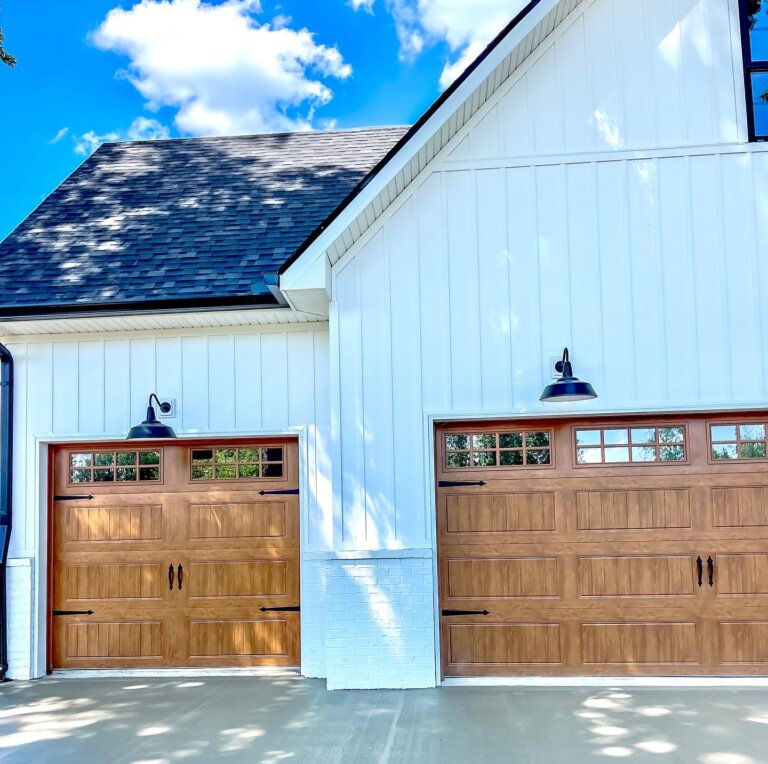The photograph is a square, low-resolution color image capturing the left side of a large, two-story house from the exterior, viewed from the middle of a concrete driveway. The scene is lit by daylight, revealing a clear blue sky with some white clouds, casting distinct shadows onto the driveway. The house's exterior is distinguished by its combination of textures: a lower section made of white-painted brick and an upper section featuring vertical white wooden slats. The slats include recessed and protruding sections that add depth to the facade. 

This section of the house appears to resemble a modern take on an old-style barn, with a traditional A-frame black roof covered in gray shingles. The structure includes a three-car garage featuring two wood-paneled doors with large windows at the top, accented by black handles. One door stands alone, separated by a small wall from a double door. Above each garage door are black metal sconce lights, designed more elaborately than typical exterior lights, casting a focused downlight in front of each door.

A distinct architectural feature is the additional vertical extension above the double garage door, marked by a horizontal seam, giving the section an additional height. Just below the roof’s peak, there is a lone window, adding a finishing touch to the building's facade. The overall design suggests a newly constructed structure, possibly meant to echo the charm and simplicity of an 1800s barn, embedded within a modern context.